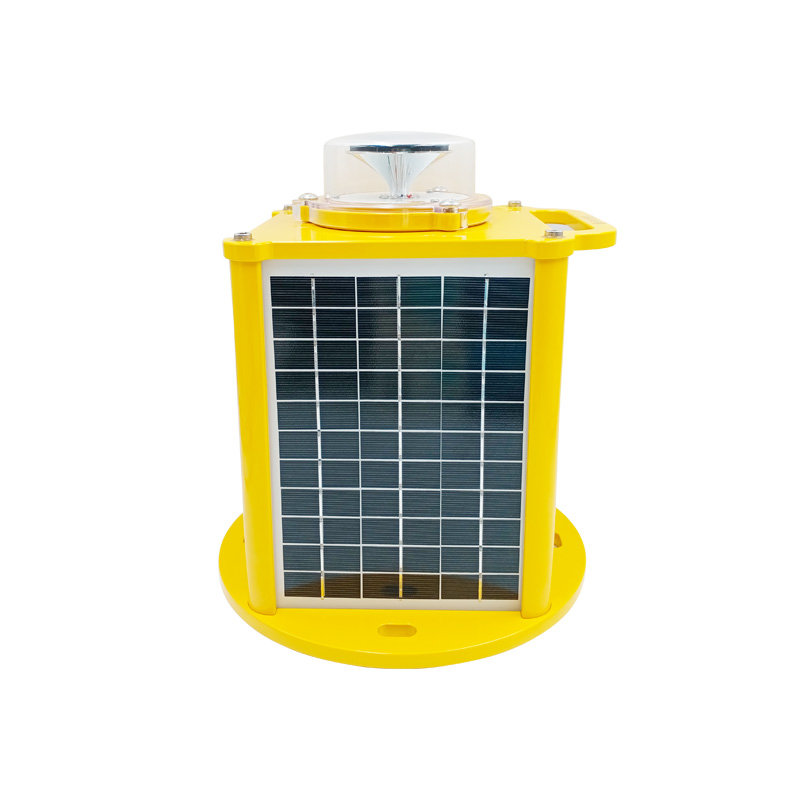The image depicts a large yellow air conditioning unit, specifically designed for outdoor placement. The rectangular body of the unit sits on a circular yellow base which features multiple small oval cutouts, possibly for securing or mounting purposes. The sides of the rectangle are adorned with white grids containing black fins. Positioned at the top is a clear plastic lid, resembling a container cover, housing a white triangular component topped with a black piece. This section may serve as a light or control mechanism. On the right side of the top, there's a handle designed for portability, allowing easy lifting and carrying by hand. The unit's top also showcases screws positioned on the edges, indicative of its structural assembly. The entire appliance exudes a robust appearance, characteristic of a major motor unit integral to an air conditioning system.